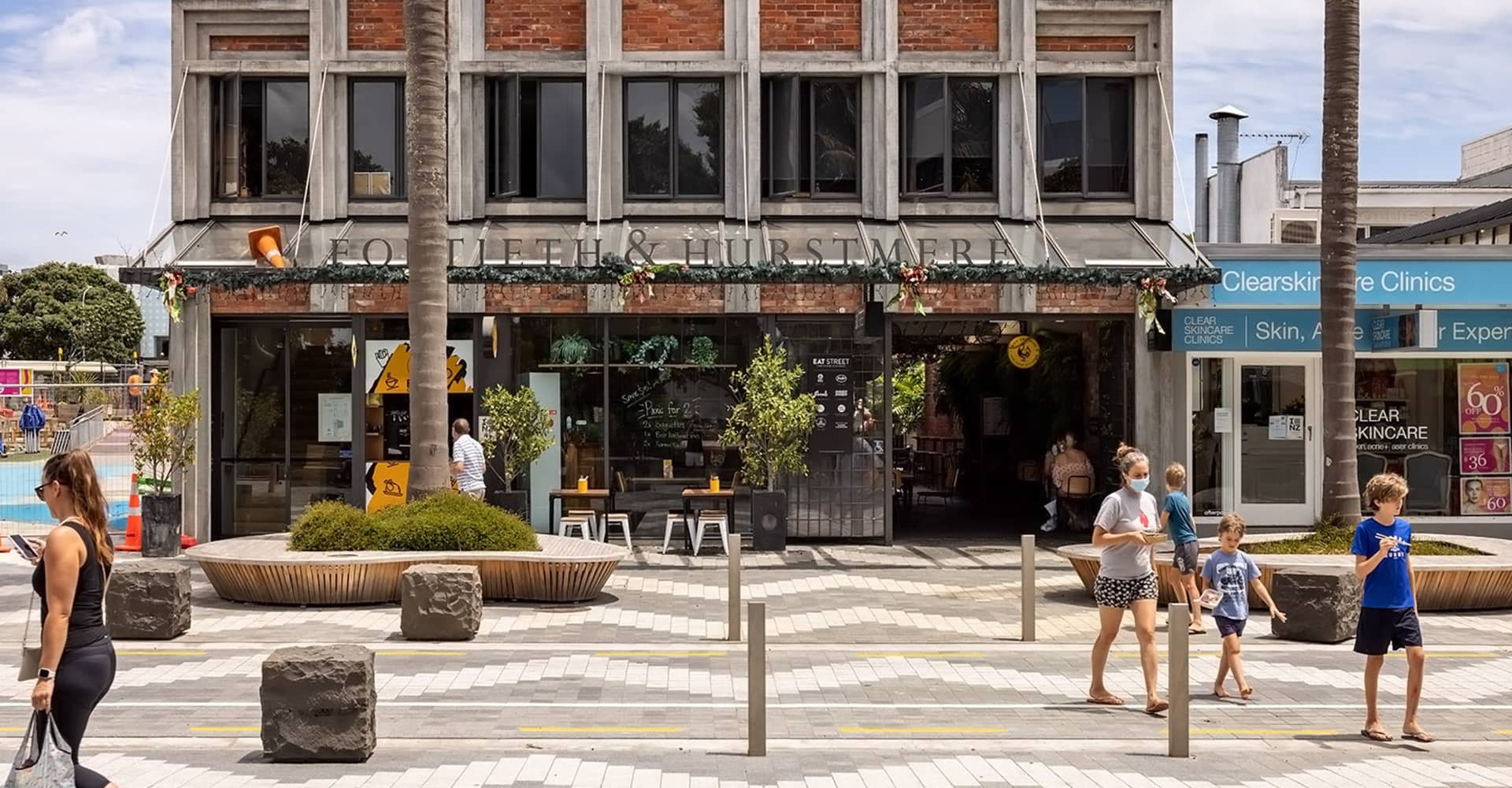This vibrant color photograph captures a bustling pedestrian plaza on a sunny day. The plaza features a geometric pattern of gray and white tiles zigzagging across the ground. Dominating the scene is a brick and concrete building with glass storefronts, prominently displaying a sign that reads either "Faux Thief and Hurstmere" or "14th Hertzmere". This building, possibly a shop or restaurant, has several tables set up outside.

Flanking the building to the right is a smaller storefront with a sign reading "Skin Care Clinic" in white text on a blue background. In the foreground, there's a tall palm tree growing within a circular wooden bench, situated amidst cube-shaped stone blocks on the walkway.

The plaza is alive with activity. To the left, a woman dressed in black, looking at her phone and carrying a bag, casually strolls by. To the right, a mother wearing a blue mask escorts four boys dressed in t-shirts, shorts, and flip-flops. Above them, a blue sky dotted with white clouds provides a picturesque backdrop to this lively street view, perhaps in a historic downtown area.